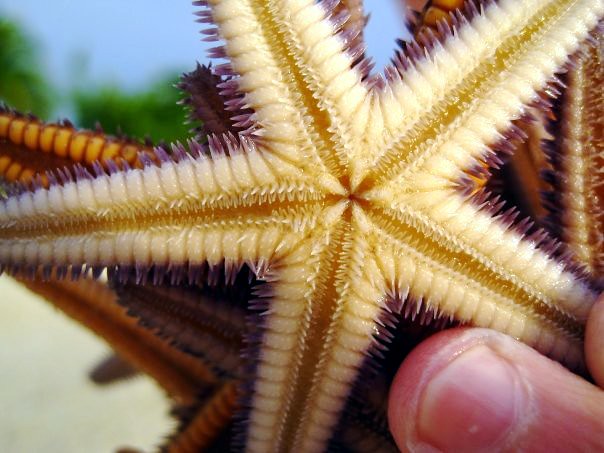In this detailed outdoor photograph, the primary focus is on a cluster of starfish held up for observation. The viewpoint showcases the underside of these starfish, with the central one displaying a light yellow color accented by dark brown towards the center. Surrounding this yellowish starfish, there are two more starfish—one with a darkish purple hue and another with a dark orange tint. These starfish, identified as the two-spined sea star, feature prickly, pin-like spikes along their sides. 

The starfish are held up by a human hand, identifiable by the visible thumb and fingernail, giving a sense of scale and interaction. In the background, a blue sky and green foliage from trees are slightly blurred, emphasizing the starfish in the foreground while adding a natural setting to the composition.